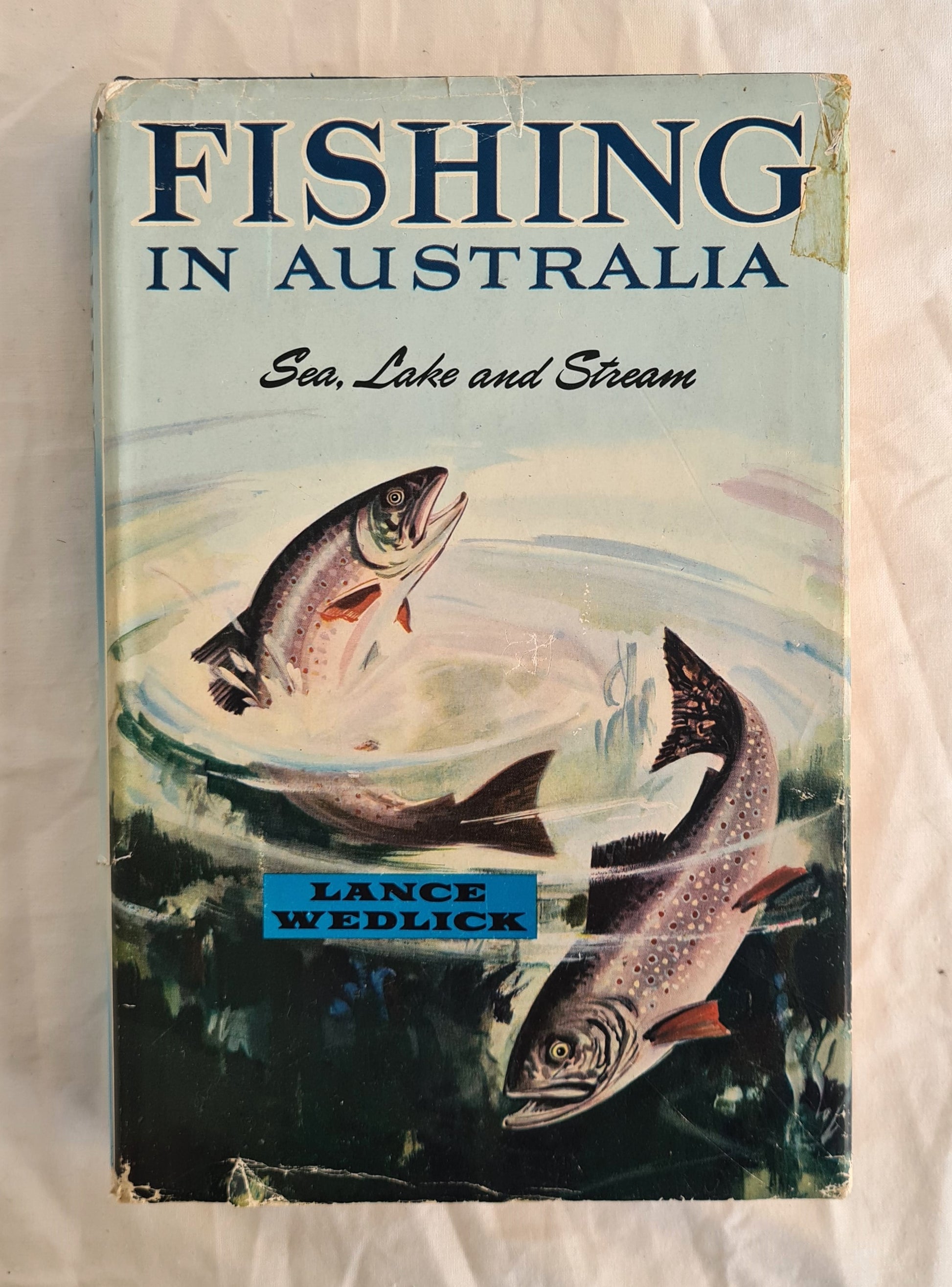This is a detailed snapshot of a worn and well-loved book titled "Fishing in Australia: Sea, Lake, and Stream" by Lance Wedlick. The book, which has a paper covering over a hardback surface, is resting on what appears to be a wrinkled white or cream-colored bed sheet or piece of paper. The cover features two trout-like fish, with one diving into the water and the other leaping out, creating visible ripples and a sense of movement. The book's blackish-gray cover is speckled with white dots and shows significant signs of wear, including creases, tears along the corners and edges, and a taped front right corner. The title text is rendered in a combination of navy blue and black.